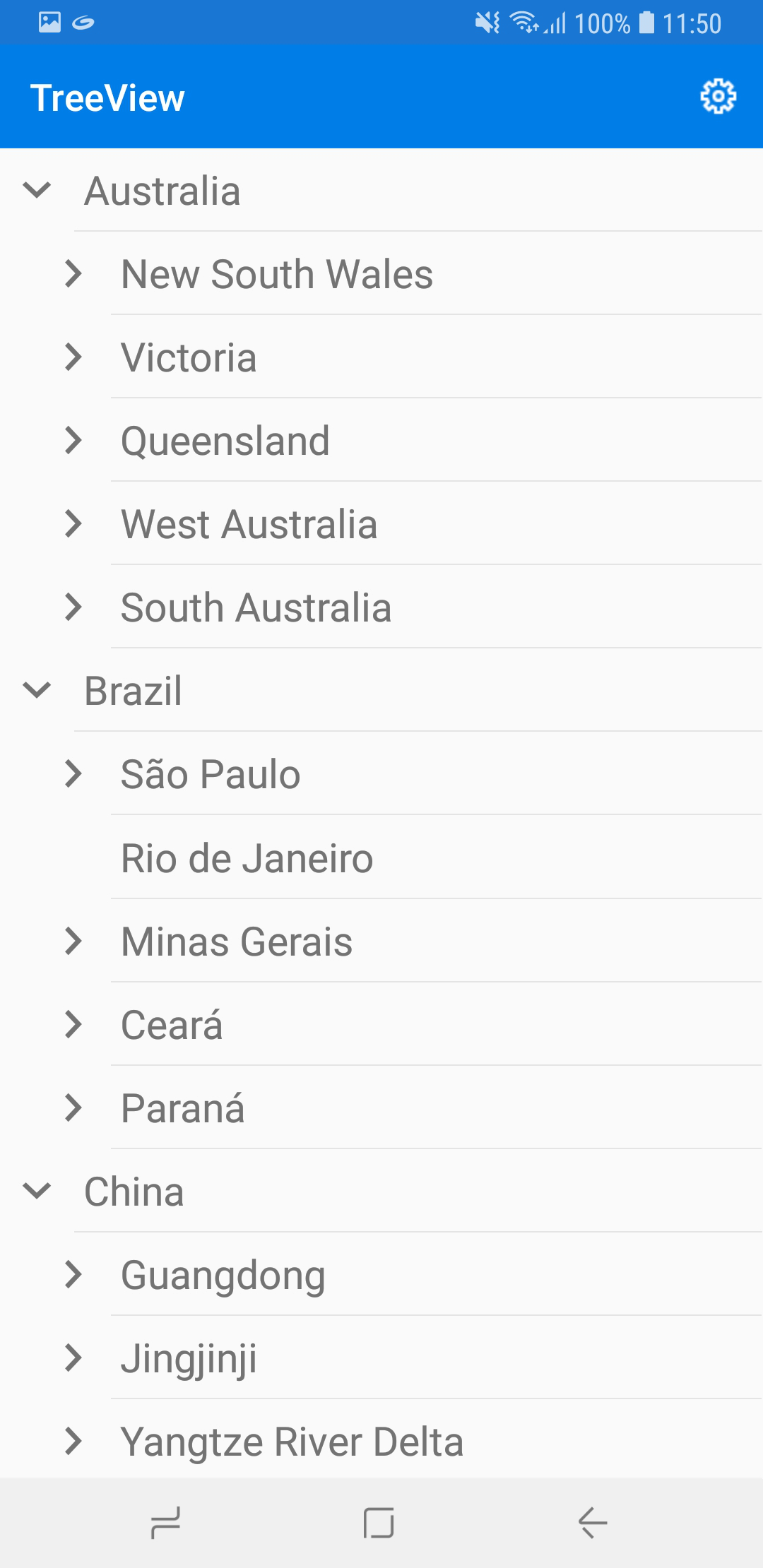A screenshot of an unidentified application displays various elements on its user interface. At the very top of the screen, there's a medium-colored status bar showing an image icon, service signal icons, a battery icon at full charge (100%), and the clock indicating 11:50. 

Below this, a lighter, thicker navigation bar features a settings gear icon on the right side and the label "TreeView," denoted in camel case, on the left.

The main portion of the screen is divided into sections representing different regions and their associated options. The first section is labeled "Australia," with a downward arrow indicating it is expandable. Nested under it are five lines, each with a right-facing arrow: New South Wales, Victoria, Queensland, West Australia, and South Australia.

The next section is for "Brazil," which is already expanded, displaying its nested options. São Paulo has a right-facing arrow next to it, while Rio de Janeiro does not have an arrow. Below these, Minas Gerais, Sierra, and Parana each have right-facing arrows.

Underneath the Brazil section is "China," also with a downward arrow. When expanded, it shows three options: Guangdong, Xinjiang, and Jiangxi River Delta, all with right-facing arrows.

At the bottom of the screen, there's an icon resembling a parallelogram with two squares inside it, next to the standard navigation buttons (a square button and a back button) typically found on a smartphone.